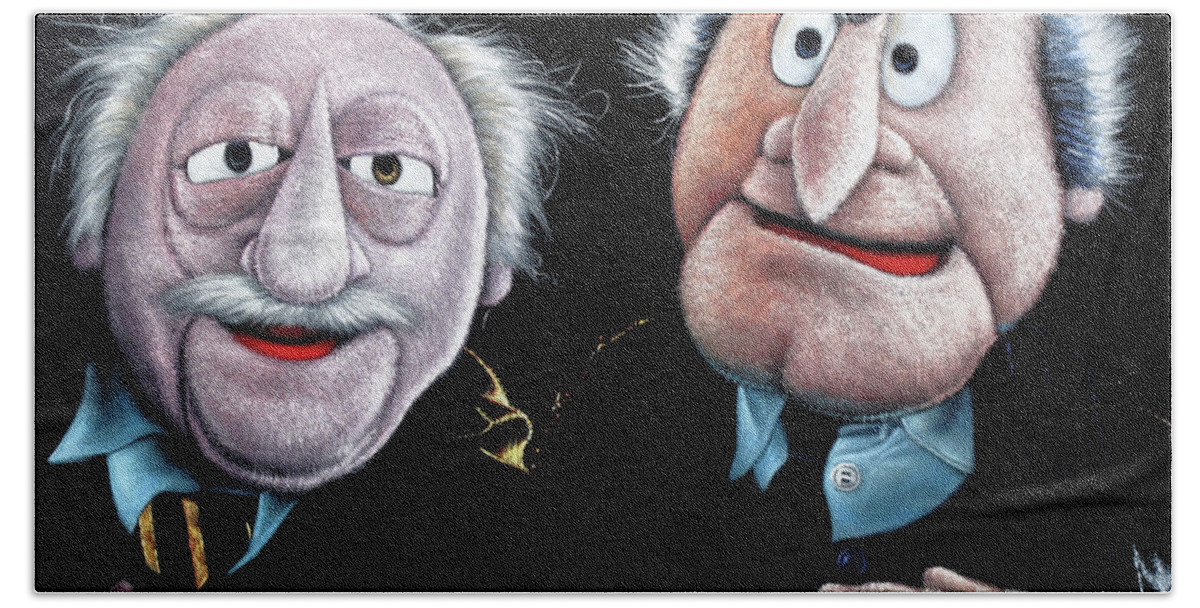The image is a detailed, color drawing depicting the two iconic old men Muppets from The Muppet Show, who are usually seen in the balcony. Their appearances are highly exaggerated and cartoonish, with a focus on their distinct facial features. Both characters have large, globular eyes, big noses, and silly, expressive faces that capture their comical essence. The Muppet on the left has gray, wild, unruly hair, a white mustache, and grayish skin. He wears a blue collared shirt, a black suit jacket, and a black and gold tie, with a smile that reveals a red mouth. The Muppet on the right, in contrast, has similar unruly gray hair but no mustache. His peach-colored skin contrasts with his white eyes and black pupils, and he sports a manic expression with his mouth open, showing the red inside. He is dressed in a blue shirt, a black necktie, and a black coat. The entire scene is set against a stark black background, enhancing the vivid and almost photorealistic appearance of the characters, though it is clearly a professionally done drawing or painting that meticulously captures the texture and essence of these classic Muppet characters.